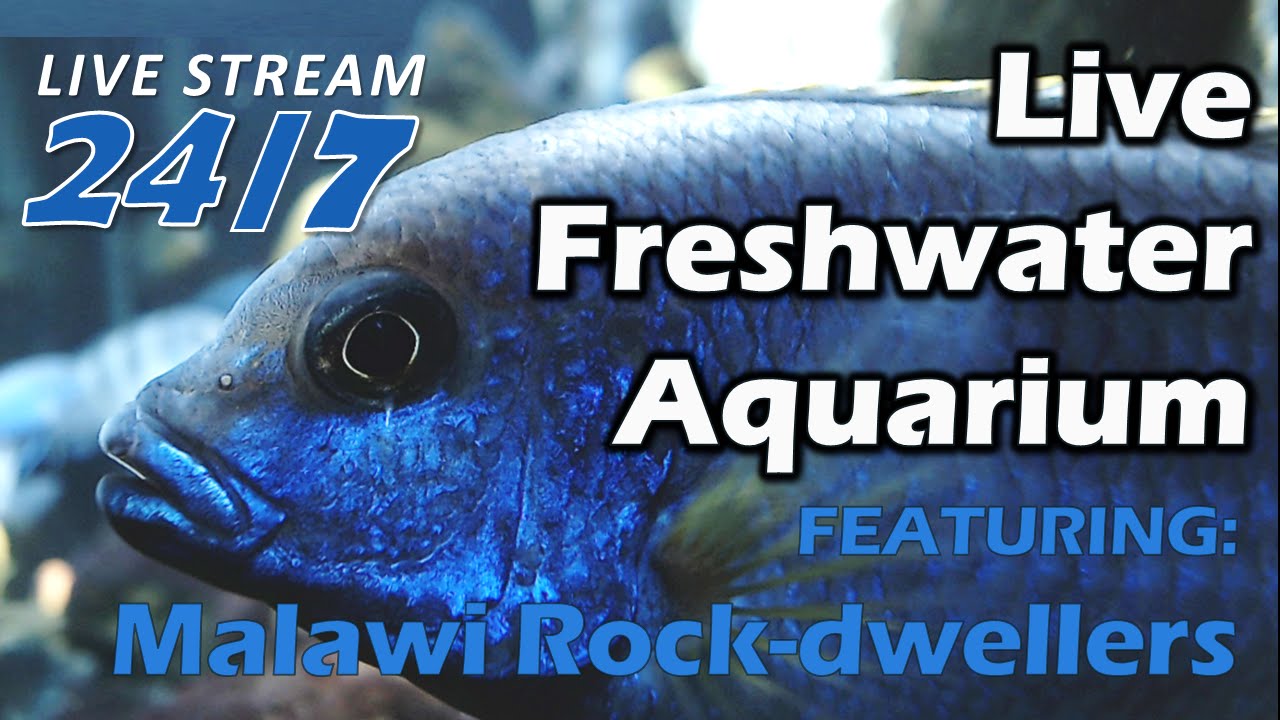This image is an advertisement for a live freshwater aquarium livestream, designed in soothing tones of blue and white. Dominating the background is a close-up photograph of a large, vibrant blue fish, possibly a Malawi Rock Dweller. The fish exhibits remarkable detail, including its sparkling, bioluminescent-like blue scales, a big black round eye, and hints of green or yellow on its fins. The overall setting is within an aquarium, with a diffused, faded background that accentuates the fish's striking appearance.

Text elements are strategically placed across the image. In the upper left corner, in a mix of blue and white text, it reads "Livestream 24-7." On the right side, in white print outlined in black, it states "Live Freshwater Aquarium" with smaller blue text underneath specifying "featuring Malawi Rock Dwellers." The text is thoughtfully positioned so as not to obscure the fish’s intricate details, allowing viewers to appreciate its fins, scales, mouth, and lips. The composition of the image is calming, with the blue tones enhancing the serene, underwater atmosphere.